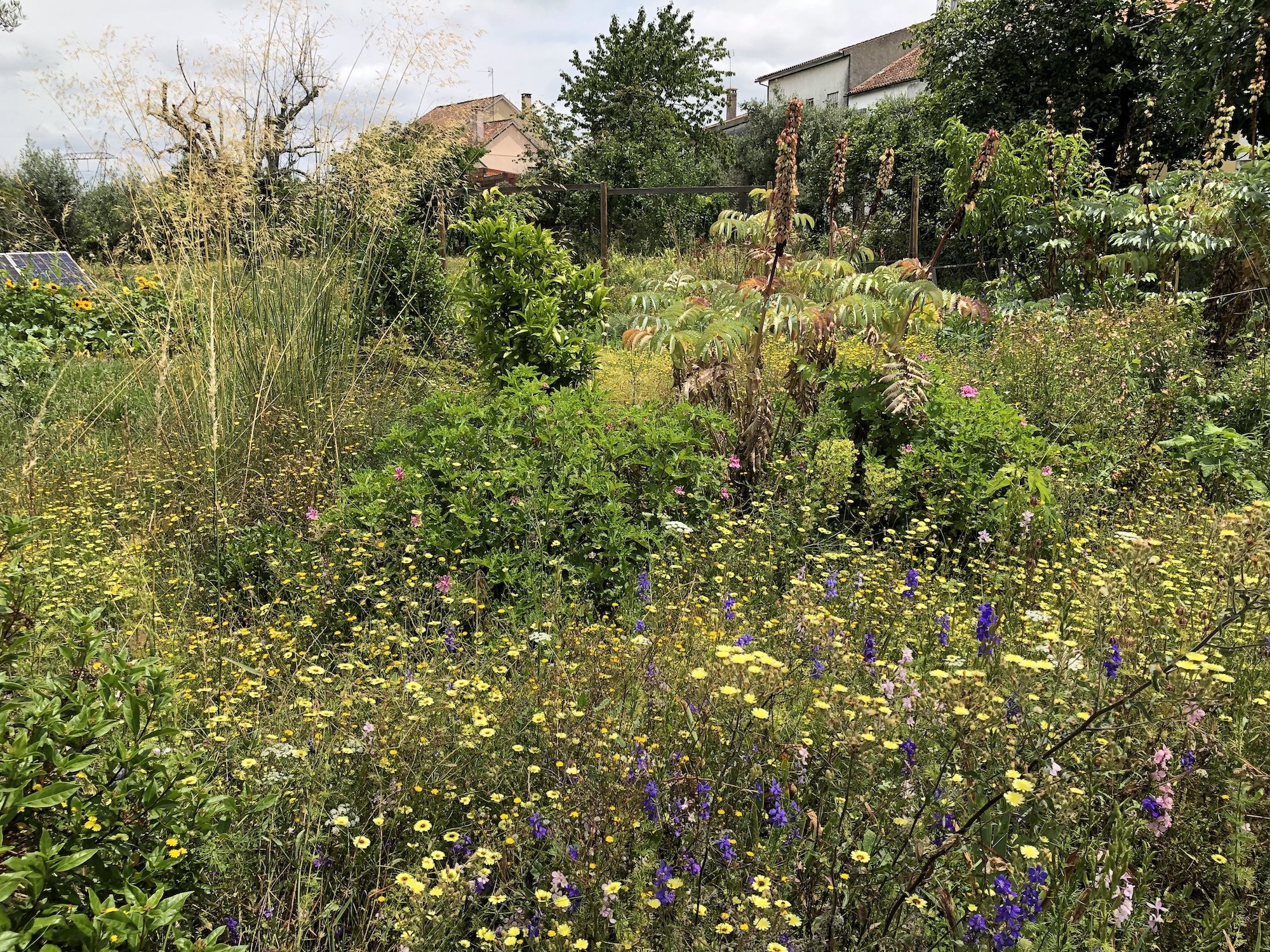An outdoor scene featuring a densely overgrown garden filled with tall grasses, an abundance of wildflowers in hues of purple, yellow, and pink, and various unruly bushes. Among the vegetation, there are a few blooming weeds and some branches from a dead tree jutting out. The overgrowth extends to trees and hedges, which obscure most of a building situated in the background, possibly a house. A fence separates the garden from a neighboring property. The sight of this vivid yet untamed garden, with its mix of colorful flowers and neglected greenery, gives an impression of natural, albeit chaotic, beauty.